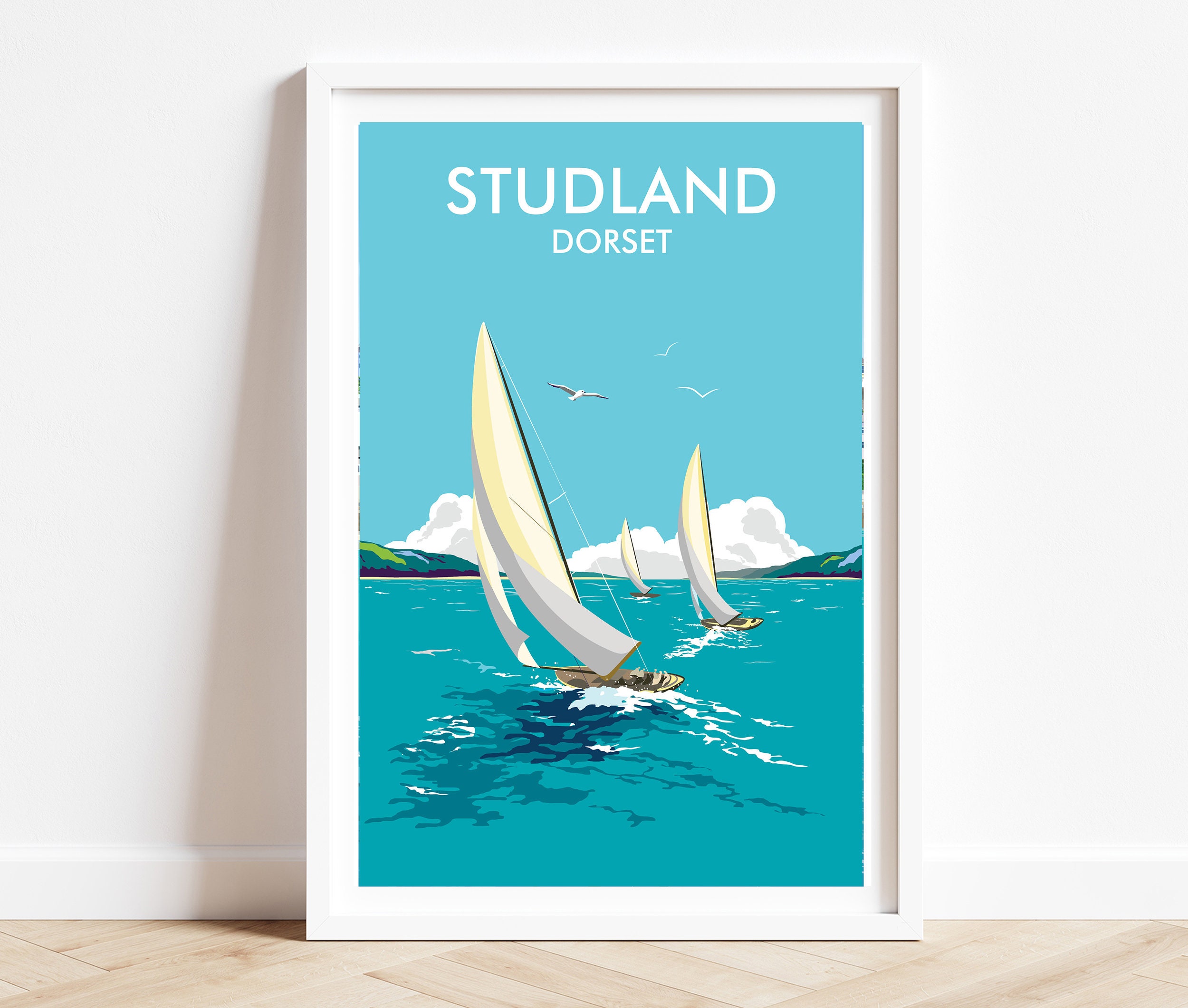The color photo captures a white-framed painting leaning against a white wall, set on a herringbone-patterned, light-tan, wooden floor. The painting depicts a serene coastal scene titled "Studland Dorset," written in capital, thin block font at the top in the light blue sky. The sky is interspersed with low, fluffy white clouds and three seagulls, one of which is in clear focus while the others appear as mere white lines. The turquoise blue water below is detailed with darker blue shadows and frothy white waves, enhancing the sense of movement among the three sailboats. The boats, with their tall white sails held aloft by green masts, appear to be swiftly navigating the waters, creating dynamic waves and splashes around them. In the distance, green hills rise subtly against the horizon, adding depth to the tranquil yet lively maritime scene.